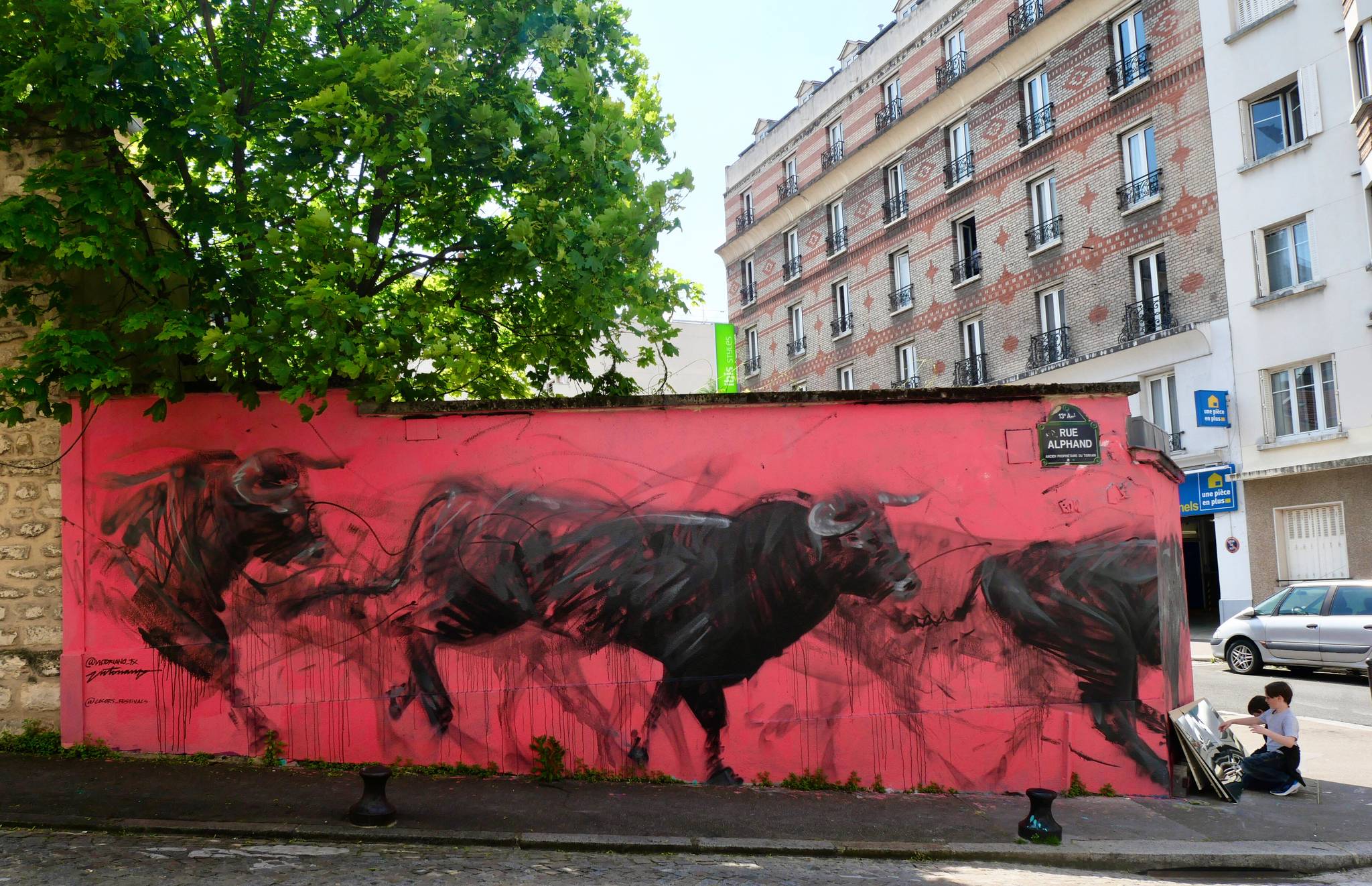The image captures a bustling city corner bathed in bright, sunny weather with a vivid blue sky. Dominating the scene is the side wall of a building painted in a striking deep coral hue, adorned with a vibrant mural that immediately draws the eye. The mural depicts three bulls in motion, painted in black with greyish horns. The artistic strokes create an impression of movement, with each bull partially depicted—the lead bull showing just its front half, the middle bull fully visible, and the trailing bull displaying only its hind part. The bulls appear to be charging from left to right off the mural, enhanced by smudgy patterns that suggest additional bulls in the background.

Above the mural is a street sign that reads "Rue Alphand," hinting that the location might be in France. Flanking the mural on the left, a large, round green tree adds a touch of nature to the urban landscape. In the background, the street extends, lined with older apartment buildings characterized by a mix of architectural details—grey with red brick accents, white windows, and black wrought iron railings. Adjacent to these buildings, there's a four-story building likely used as apartments, with open windows and wrought iron guardrails.

The scene also features a four-door silver car parked on the street and a green banner hanging from one of the red and brown brick buildings. On the sidewalk at the mural's edge, two children are kneeling, engaged with paintings propped against the wall. One child wears a grey shirt and black pants. The entire scene conveys a lively, picturesque urban environment with a blend of artistic flair and everyday life.